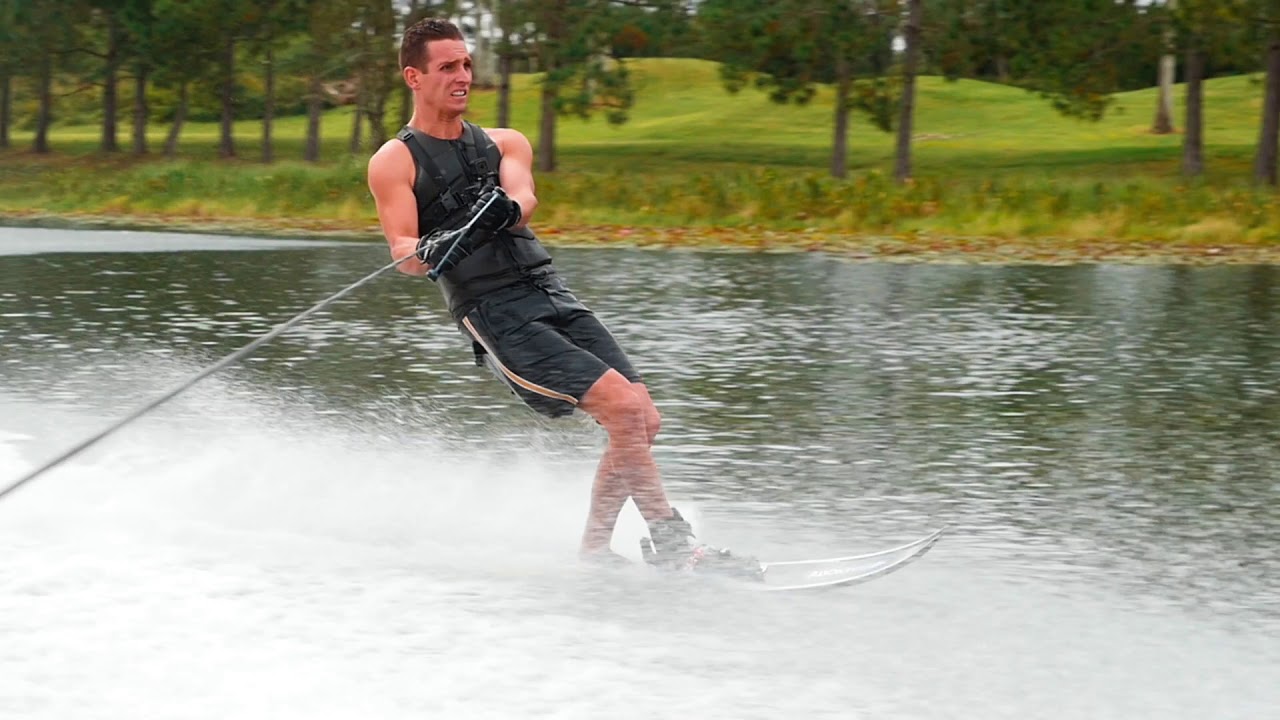A man is captured in an intense moment of water skiing on a murky, green-colored lake. He is slaloming on a single ski with both feet secured, gripping the tow rope, which trails off to the left, attached to a boat not visible in the image. His muscular arms and black tank top, paired with long black shorts featuring a side stripe, highlight the physical exertion required for the sport. His face is strained and focused, showing immense concentration and effort. Water sprays dramatically around him from the motion of his ski cutting through the lake. In the background, marshy grasses and rich green trees tinged with orangey-red hues frame the setting. Beyond the shoreline, a freshly mowed green lawn, resembling a golf course, stretches out with a distant house perched on a hill. The lighting is flat, suggesting the sun is obscured by clouds, casting a subdued light over the entire scene. The image captures the solitary man's vigorous and focused endeavor on the serene lake.